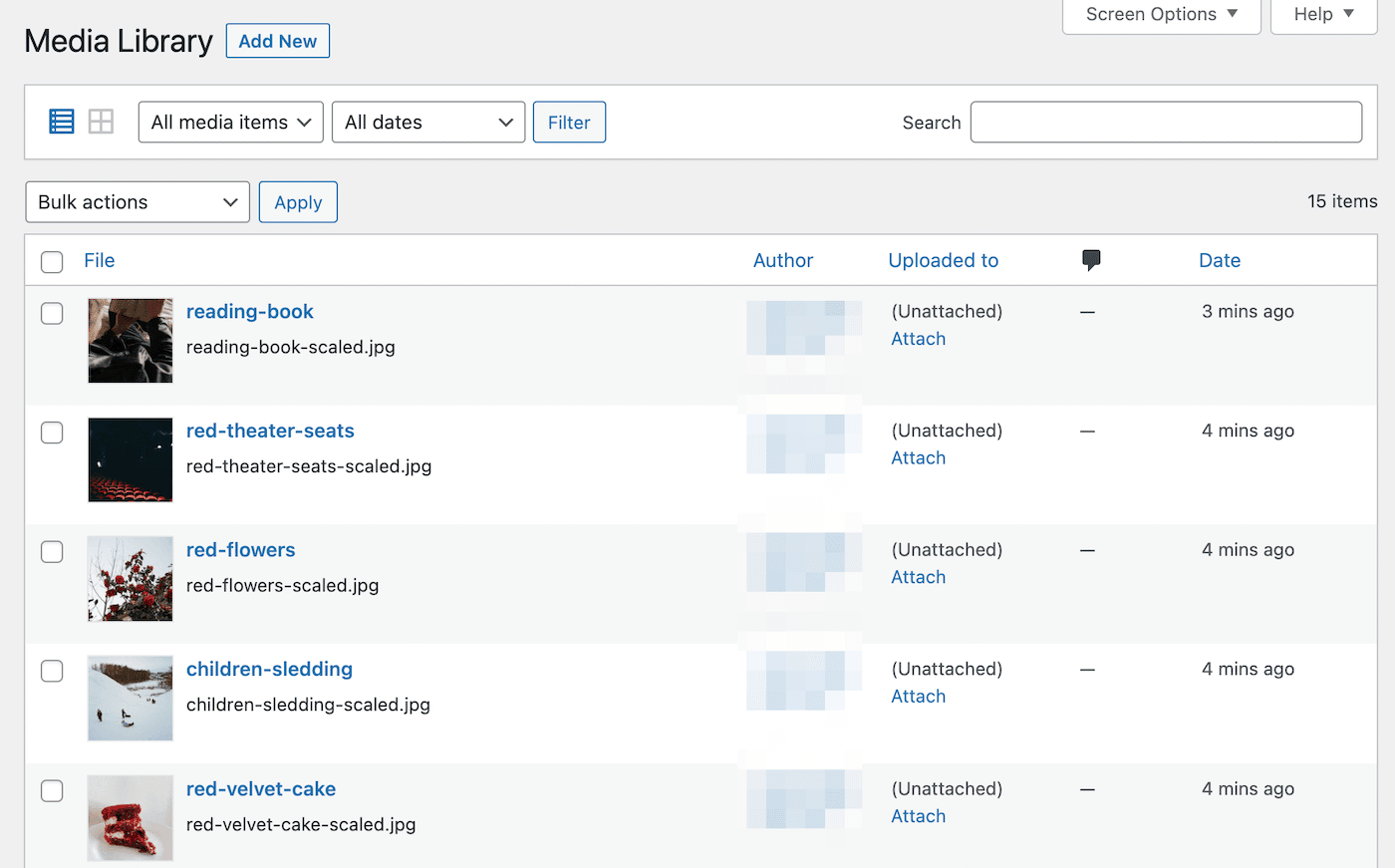The screenshot captures a detailed view of a media library interface. Dominating the scene is a large gray rectangle, indicative of a typical digital workspace. In the top left corner of this interface, the title "Media Library" is prominently displayed in black text. Adjacent to this title, towards the right, is a functional button labeled "Add New."

Positioned in the top right corner of the image, there are options and help modules. Below this, a white horizontal bar hosts several interactive elements: drop-down menus labeled "All media items" and "All dates," a "Filter" button, and a search bar positioned on the far right.

Beneath the horizontal bar, there is a secondary menu on the left side featuring a drop-down option titled "Bulk Actions" accompanied by a gray button named "Apply."

The main section of the interface showcases a list of media items, indicating there are a total of 15 items in the library, with five being currently visible. Each item is categorized under headers like File, Author, Uploaded to, and Date.

The first item listed is titled "Reading Book," marked as unattached, and uploaded three minutes ago. Following this, "Red Theater Seats" is another unattached item uploaded four minutes ago. "Red Flowers," featuring an accompanying image of red flowers, is similarly unattached and uploaded four minutes prior. "Children's Sledding" displays an image of people sledding in white snow and is unattached as well, uploaded four minutes ago. The final visible item is "Red Velvet Cake," rounding out this portion of the media library.

This comprehensive look at the media library offers a clear insight into the structure and recent additions to the repository.